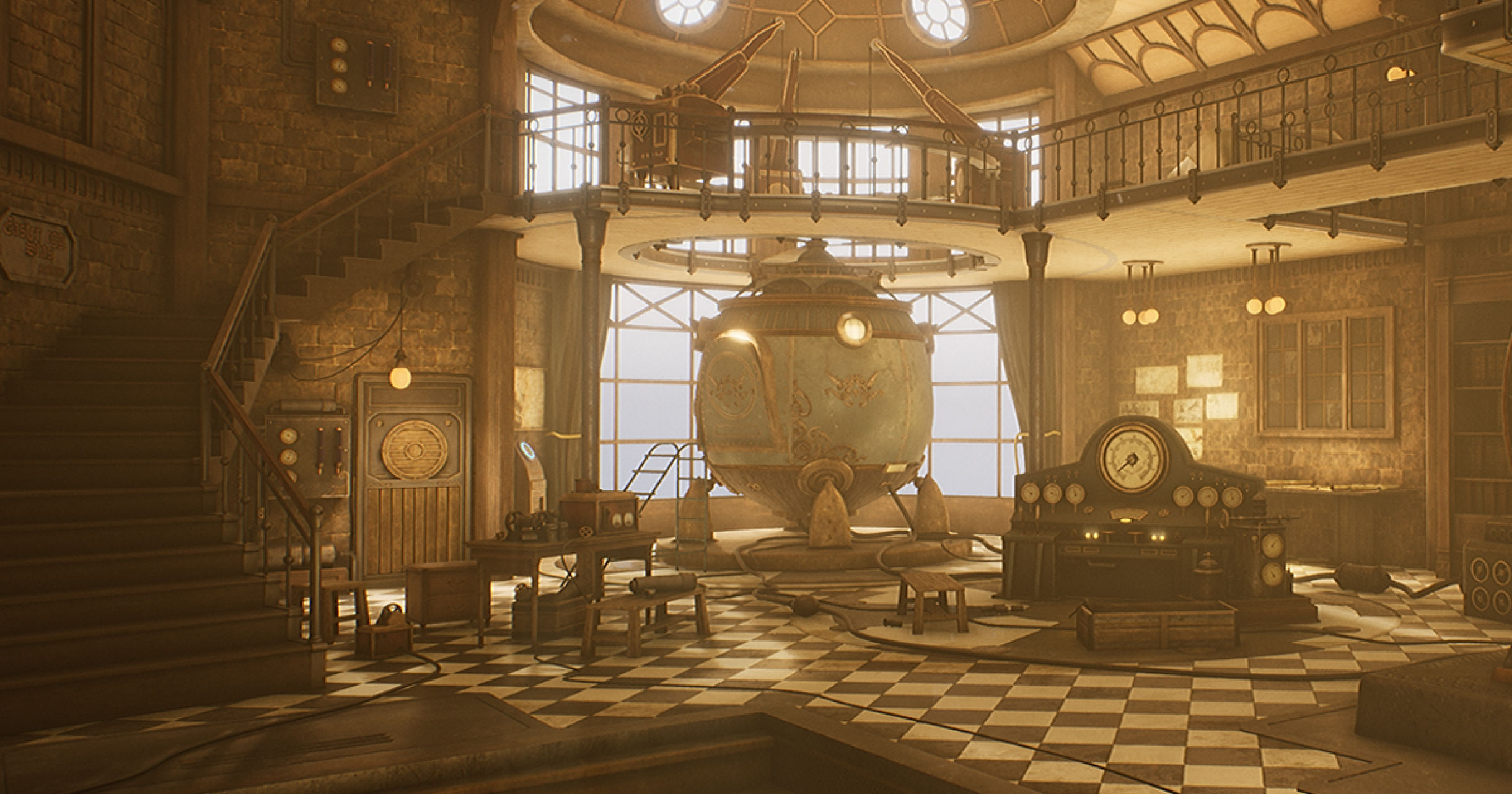This photograph captures an elaborate and expansive two-story room, likely within a home, characterized by its rich brown and tan hues. A prominent feature of the room is a striking black-and-white checkered tile floor. Dominating the center is a massive, ornate contraption resembling a cauldron or intricate machine, embellished with blue and gold designs. This central piece extends upward, its tip piercing through a hole into the second floor. 

The second story hosts an observatory with a large picture window stretching to the ceiling, letting in ample natural light. A balcony lines the right side of the second story, while a grand, curved staircase on the left ascends to the upper level. Adjacent to the main contraption is a detailed control panel with various instruments. Additionally, a small desk with more contraptions is situated nearby. The ceiling is adorned with skylights that illuminate the cauldron-like machine, adding to the room's intricate and elaborate ambiance.